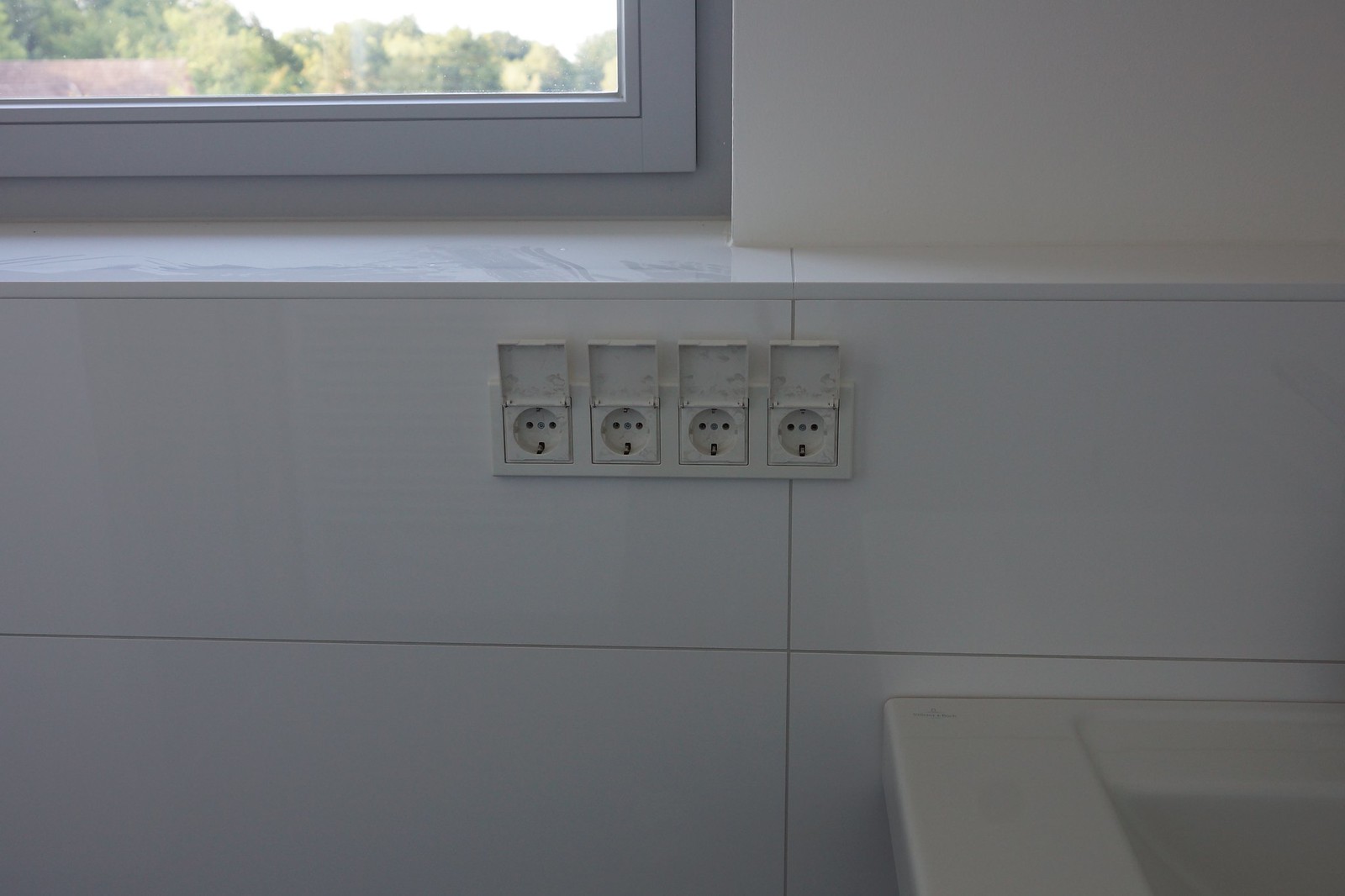This detailed photograph captures a white room with a set of four horizontal power outlets prominently featured in the center. These outlets are distinctly non-American, likely European, as they each have three aligned holes—the middle of which appears to be filled in or lighter in color—along with square protective lids that are flipped up. The outlets, intended to protect the plugs when not in use, have a noticeable gray-beige staining, suggesting they haven't been cleaned or maintained regularly. Positioned below a ledge, the outlets are set against a bright white wall made of shiny tiles or paneling.

In the upper left corner, part of a window is visible, outlined by a white frame. Through the window, daytime light streams in, revealing green trees and the edge of a distant brown tiled roof. The ledge above the outlets, which runs beneath the window, is cluttered with dust and fingerprints, indicating it hasn't been cleaned recently.

In the bottom right corner of the image, a hint of either a bathtub or a sink can be seen. This fixture is white and dips inward, further suggesting a bathroom setting. Overall, the room offers a striking contrast between its intended cleanliness and the subtle signs of neglect.